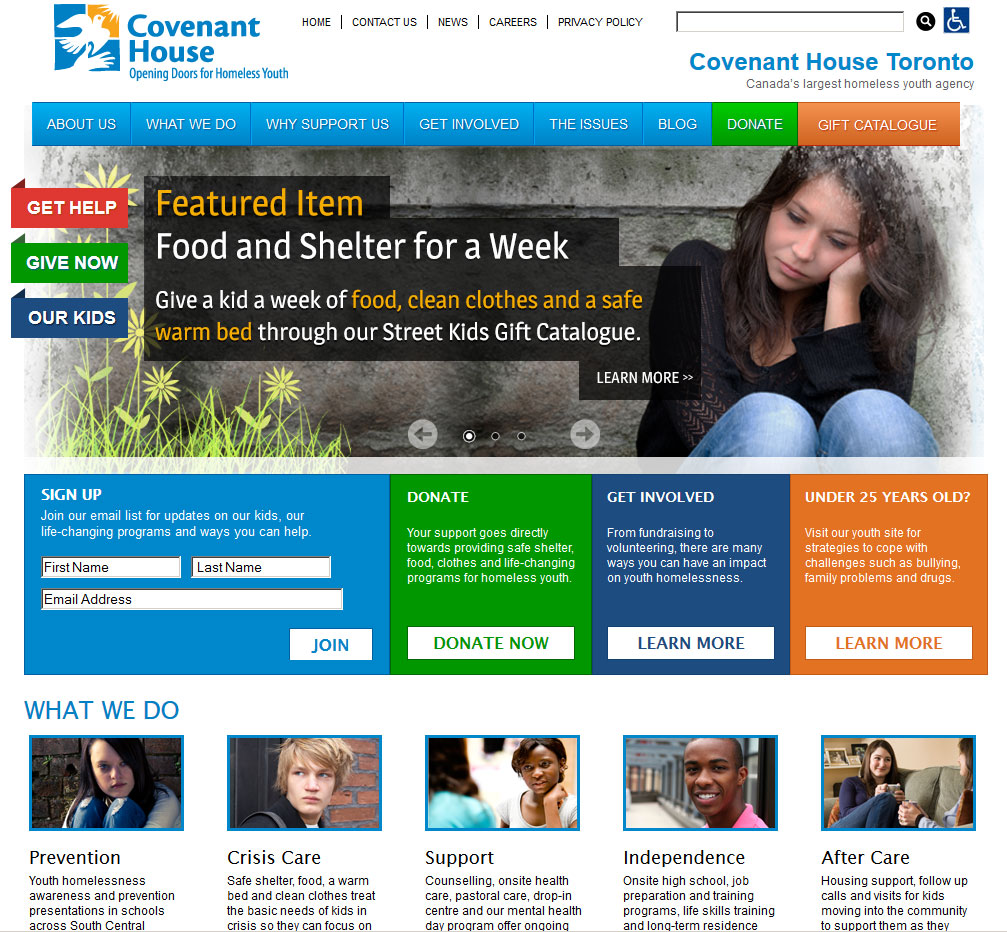This is a detailed caption for the image provided:

---

A screenshot of the Covenant House website, a sanctuary for homeless youth located in Toronto, Canada, is prominently displayed. The website header includes navigation links like "Home," "Contact Us," "News," "Careers," and "Privacy Policy." Below the header, a banner is adorned with site-wide navigation options: "About Us," "What We Do," "Why Support Us," "Get Involved," "The Issues," "Blog," "Donate," and "Gift Catalog."

The centerpiece of the banner features a poignant image of a young girl with brown hair, seated against a wall. She wears a black sweater and blue jeans and appears visibly distressed with her head resting on her hands. To the left of her image, an illustration of grass adds a touch of artistic flair.

Beneath this emotional banner, the website is segmented into four interactive boxes:
1. "Sign Up" – Offering visitors an opportunity to join the organization's mailing list.
2. "Donate" – Directing users to a donation page to support homeless youth.
3. "Get Involved" – Guiding visitors on how to contribute through volunteering or other means.
4. "For Under 25" – Providing vital information and resources for youth in need.

Following these sections, five additional boxes describe the organization's key initiatives:
1. "Prevention" – Highlighting efforts to prevent youth homelessness.
2. "Crisis Care" – Emphasizing immediate support services for youth in crisis.
3. "Support" – Showcasing ongoing assistance provided to those in need.
4. "Independence" – Detailing programs aimed at fostering self-sufficiency among the youth.
5. "Aftercare" – Focusing on long-term support for those transitioning out of homelessness.

Each of these sections includes visuals of individuals engaged in these various programs, reflecting the diverse efforts of the Covenant House in addressing the multifaceted issue of youth homelessness.